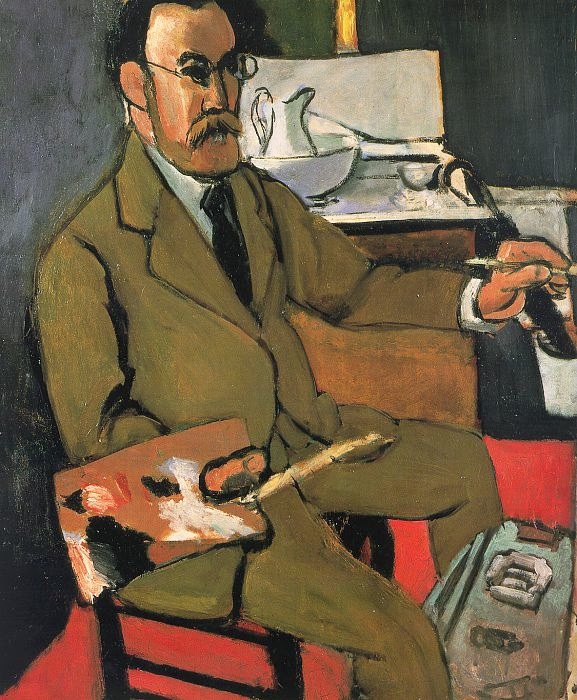This painting depicts a man who is a painter, seated in a black, four-legged chair facing the right side. The man is dressed in a brown or olive green suit with a white shirt and a black tie. He has dark, short hair, wears glasses, and sports both a mustache and a beard. The man holds an artist's palette, which contains black and white paint, in his right hand, while he paints with a brush in his left hand. Between his legs, there appears to be a bag or some form of luggage, possibly holding his art supplies, resting on a red floor. The scene behind him includes a simplistic, outlined rendering of a table with a white pitcher and bowl set against black walls, adding to the flat, two-dimensional and dramatic, bold color scheme of the artwork.